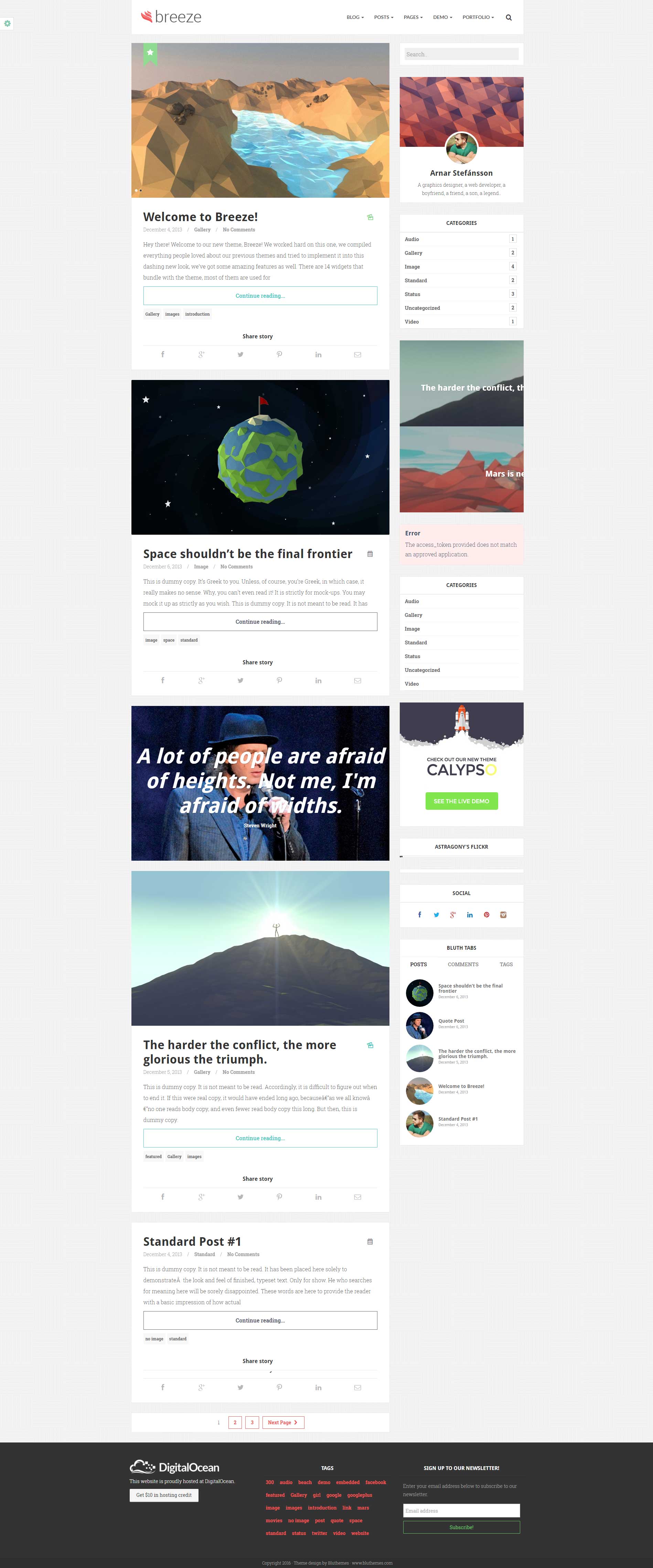The image depicts a section of a web page that features very small and challenging-to-read print. The layout is predominantly vertical, measuring approximately four times longer than it is wide. 

At the top center, there is a white bar labeled "Breeze," accompanied by six indistinct options to its right. In the left column, a series of visual and textual elements are arranged as follows:

1. **Top Section**:
   - A photograph showcasing water amidst sand dunes.
   - Beneath the photo, the text "Welcome to Breeze" followed by an unreadable paragraph.

2. **Middle Section**:
   - An image of a planet with the heading "Space shouldn't be the final frontier," followed by another illegible paragraph.
   - A square image featuring a person with a microphone and overlaid text stating, "A lot of people are afraid of heights; not me, I'm afraid of widths."

3. **Bottom Section**:
   - An image of a bright light atop a hill with a person seemingly standing in the light.
   - The caption below this image reads, "The harder the conflict, the more glorious the triumph."
   - Finally, at the bottom of the column, it says "Standard Post Number One."

On the right side, the layout includes an icon that likely represents the author or user, a list of unknown content, and additional statements that are too small to read. This detailed depiction highlights the page's intricate structure and the challenge of interpreting its smallest print.